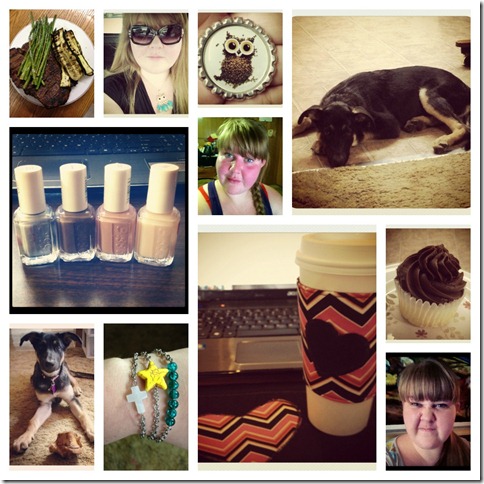The montage showcases 11 various images featuring a woman, a dog, and several products she uses. In the top left corner, a white plate displays a steak topped with asparagus and assorted fried vegetables. To its right, there's an image of the woman outdoors, donned in black sunglasses. Below, a medallion featuring an owl design appears. In the top right, a larger photo depicts a black dog resting on the ground beside a beige carpet. Leftward, a close-up of a laptop shows four beauty products in front—grayish, brown, reddish, and yellow-filled bottles. The bottom left contains another picture of the dog on the carpet. Adjacent to that, a photo of a wrist adorned with three bracelets, including a white cross, a yellow star, and turquoise stones. Nearby, a larger image captures a laptop screen with a coffee mug beside it on a wooden surface. The top right corner holds an image of a chocolate cupcake, and below it, another photo of the woman making a grimace face. The woman appears again indoors, illuminated by greenish lighting, her face visibly red, and her long blonde hair styled with bangs and a braid.